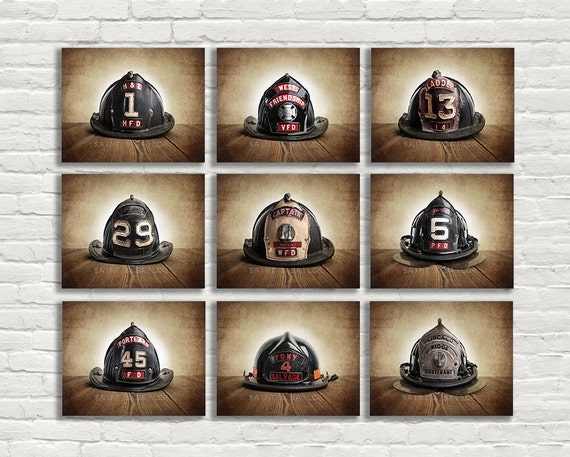The image showcases a meticulously arranged series of nine photographs, each measuring five by five inches, elegantly mounted on a white painted brick wall consisting of twenty evenly spaced rows of bricks. These photographs, captured on a wooden table with a sepia-toned background, feature an array of black fireman's helmets, each with distinct numbers, text, and insignia.

In the top row, from left to right:
- A helmet marked with H&L, number 1, and HFD (likely Houston Fire Department).
- A helmet featuring the emblem for West Friendship VFD (Volunteer Fire Department).
- A helmet labeled Ladder 13.

In the middle row, from left to right:
- A helmet numbered 29.
- The captain’s helmet, marked with number 11.
- A helmet numbered 5, with the initials PFD.

In the bottom row, from left to right:
- A helmet numbered 45.
- A helmet labeled Tony Salvage, with the mark 4.
- A helmet identified with Chicago Ridge, although the number is hard to discern.

Each photograph highlights the unique details of the fire helmets, including varying text in white, red, or gold and distinct crests, all set against the same consistent sepia-toned background and dark wooden surface. The collection offers a unified yet diverse portrayal of fireman's helmets, signifying different ranks, stations, and departments.